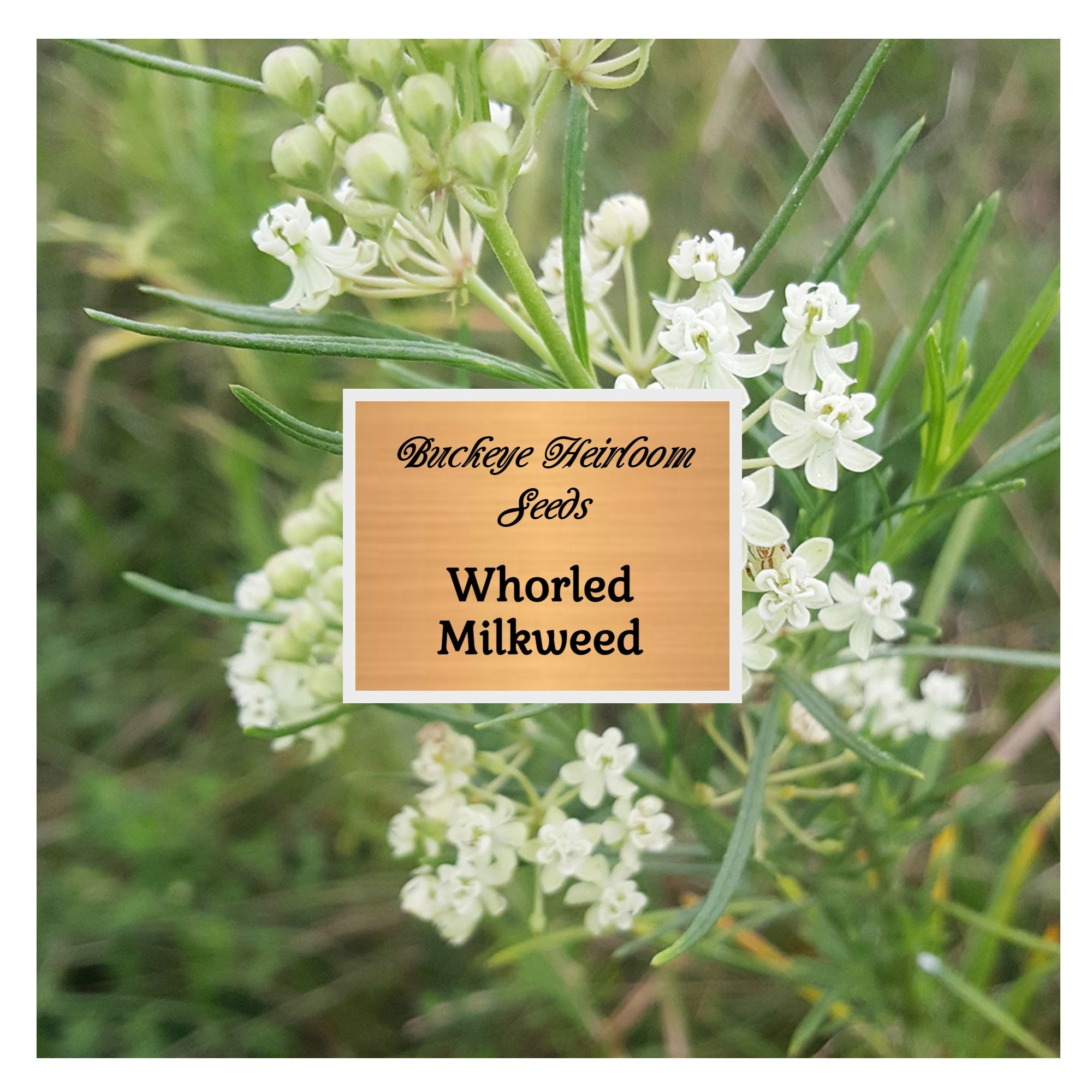This image depicts a lush outdoor scene centered on a Whorled Milkweed plant, showcasing its delicate white flowers and slender, lanceate, light green leaves. The backdrop is filled with vibrant greenery and additional plants, adding to the natural ambiance. At the center of the plant, a prominent rectangular plaque with a wood-grained yellow background and a white border draws attention. In elegant cursive script, the plaque reads "Buckeye Heirloom Seeds," while beneath in bold black type it clearly identifies the plant as "Whorled Milkweed." The flowers of the Whorled Milkweed are small, white, and numerous, with petals radiating gracefully from central stamens. This descriptive detail not only identifies the plant but also highlights its natural beauty amidst its verdant surroundings.